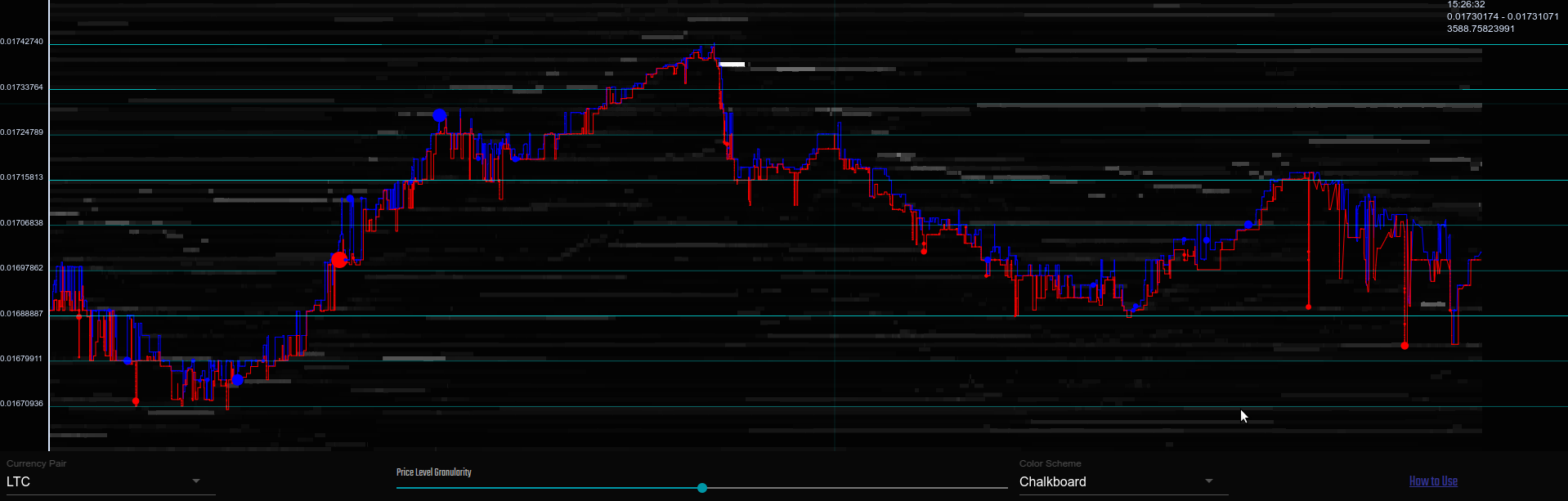This color image showcases a graph, likely from an analytical instrument or a stock chart, depicted on a digital screen with a black background. Two prominent, jagged lines—one red and one blue—extend across the graph, resembling the spiky waves of an echocardiogram. These lines start in the middle-left, dip downward, ascend to their highest point near the upper middle, and then oscillate up and down towards the right side. The graph is intersected by thin green grid lines for reference, with a particularly bright green line running near its center. On the left side, a vertical white line with tiny, unreadable labels indicates a scale of measurements. The bottom features a combination of green and white lines with the label “chalkboard.” Additional small white text is present in the upper right corner, and there is some red text in the lower right corner, both difficult to read. This detailed graph, with its complex web of colors and lines, is clearly intended for in-depth data analysis.